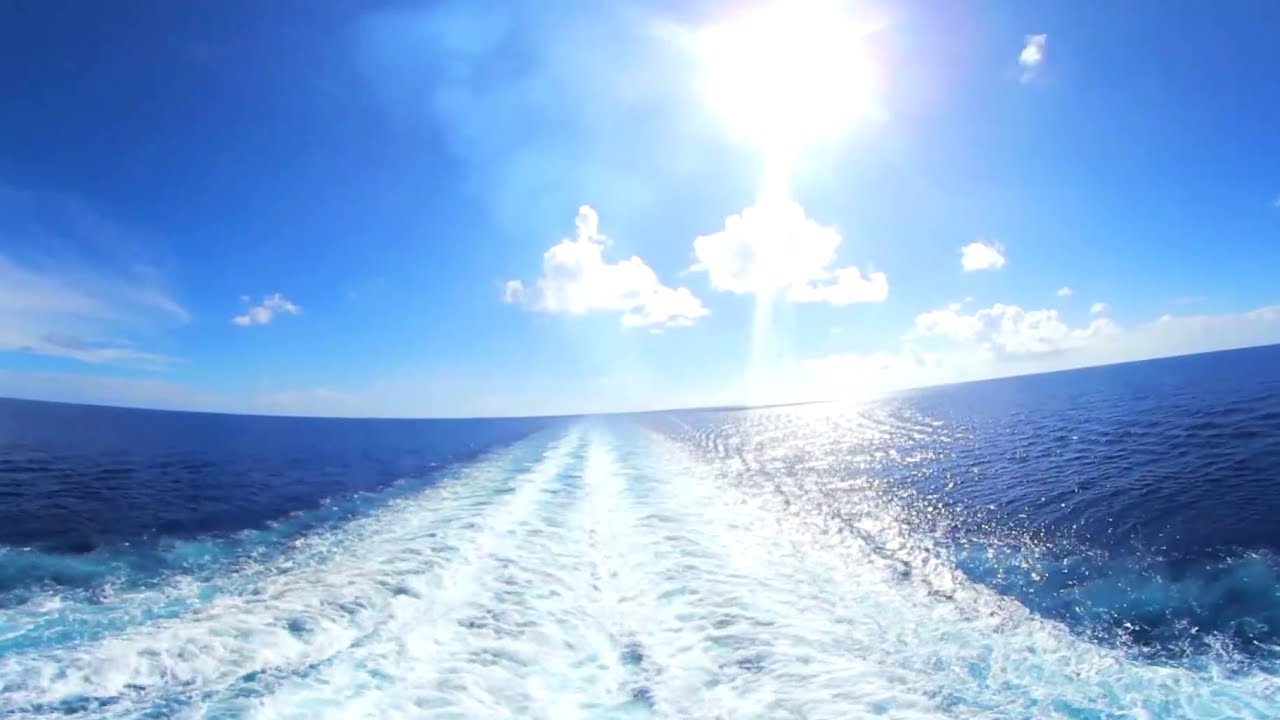The image showcases a serene outdoor scene in the middle of a vast ocean, split evenly between clear blue water and a bright, almost cloudless sky. The centerpiece of the image is a trail of foamy white waves created by a boat, giving the impression that the viewer is seated at the back of the moving vessel. To the left and right of this turbulent trail, the water transforms into deeper, stiller blue expanses. The horizon, with its slight curvature, divides the scene, with big blue skies dotted with minimal yet striking puffy white clouds, particularly clustering in the middle and on the right-hand side of the image. Wispy clouds are present toward the top and the left side, while the brilliant sun shines down, reflecting its light off the water on the right. The scene is devoid of any people, animals, or objects, emphasizing the vast, undisturbed beauty of the ocean and sky.